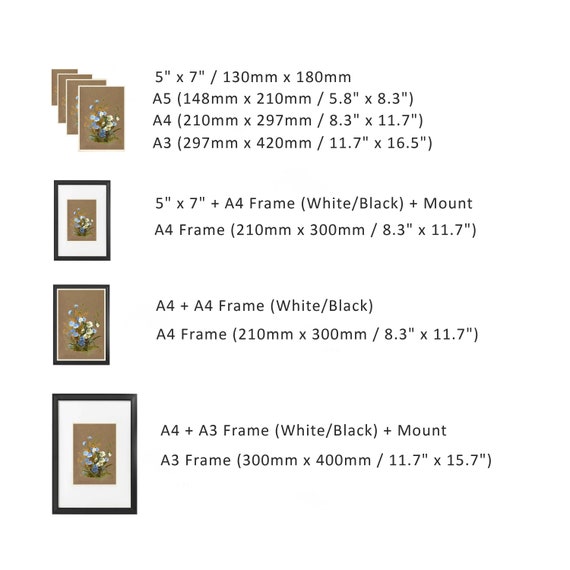The image appears to be a page from a catalog or website showcasing various picture frames. It features four different frame sizes, each depicted on the left side with a detailed description on the right. The frames range in size from 5 inches by 7 inches up to 11.7 inches by 16.5 inches and are categorized by their compatible sizes: A5, A4, and A3. 

1. The first option includes a set of four frames with sizes varying between 5 inches by 7 inches and larger dimensions. 
2. The second option presents a single black frame measuring 5 inches by 7 inches with a white mount.
3. The third option highlights an A4 frame with a black frame and a slender white mount.
4. The fourth option shows a larger frame, specifically 11.7 inches by 16.5 inches, again featuring a black frame with a white mount.

All frames display an identical image of a bunch of flowers in a vase or bucket, set against a brown background. This page effectively details the frames' dimensions, materials, and visual presentation to aid in selection.